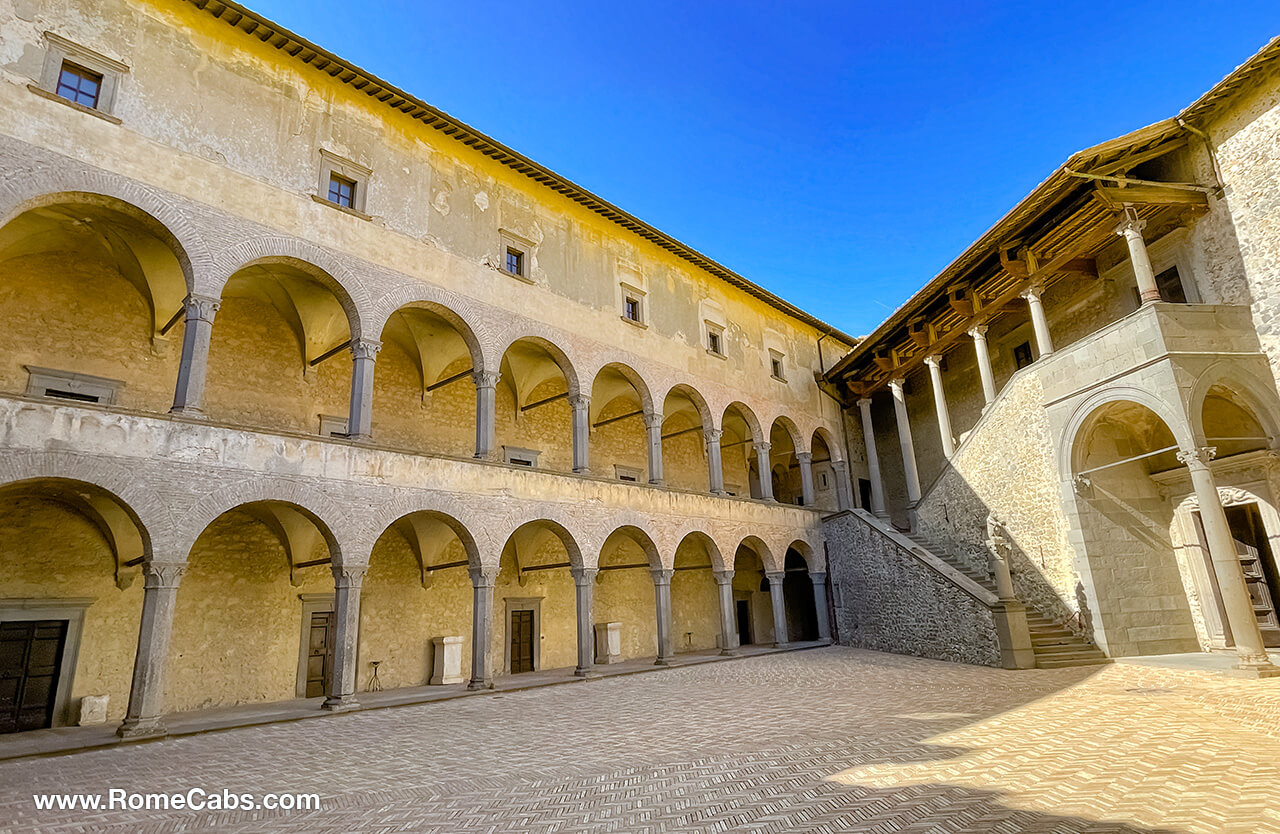The image depicts a beautifully restored historic courtyard, likely situated in Rome, as indicated by the text "www.romecabs.com" in the bottom left corner. The courtyard is framed by ancient stone buildings, showcasing classic Roman architectural elements. The structure spans three stories, with the bottom two floors adorned with Roman-style columns supporting multiple archways. Each archway houses a small door, hinting at the building's past residential or communal use. The top floor features numerous windows, suggesting thoughtful restoration with modern amenities.

The courtyard’s ground is paved in cobblestone, enhancing its timeless aesthetic. A prominent stone staircase elegantly curves up to the second floor, allowing access to the upper levels. Within the courtyard, the space feels expansive and open, punctuated by a statue atop one of the columns, though the details of the statue are indistinct. The vibrant blue sky above forms a striking triangle, contrasting with the aged stone, connecting the viewer to the ancient splendor of the scene. The combination of classical columns, arched walkways, and well-preserved masonry reflects a site of significant historical and architectural value.